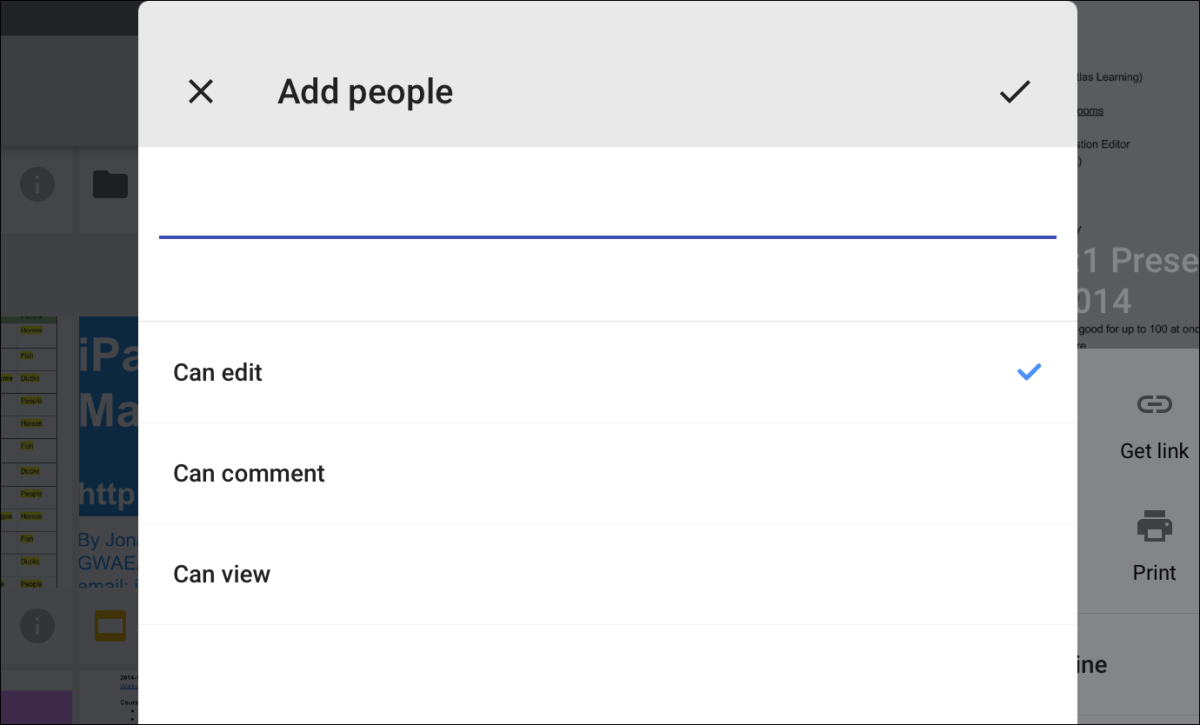The image depicts a cluttered web interface dominated by multiple overlapping pop-up windows. The background layer appears to be a webpage, though it's mostly obscured and characterized by extensive white space, making it difficult to identify its specific content. The middle layer features a dialog window offering several options, including "Print" and "Get Link," which suggest tools for managing or sharing online content. The topmost layer is another pop-up window titled "Add People," indicating a Google document interface. This pop-up facilitates adding collaborators and setting permissions, such as "Can edit," "Can comment," and "Can view." The current setting shows that users being added can edit the document, suggesting an active effort to expand collaborative access to the document.